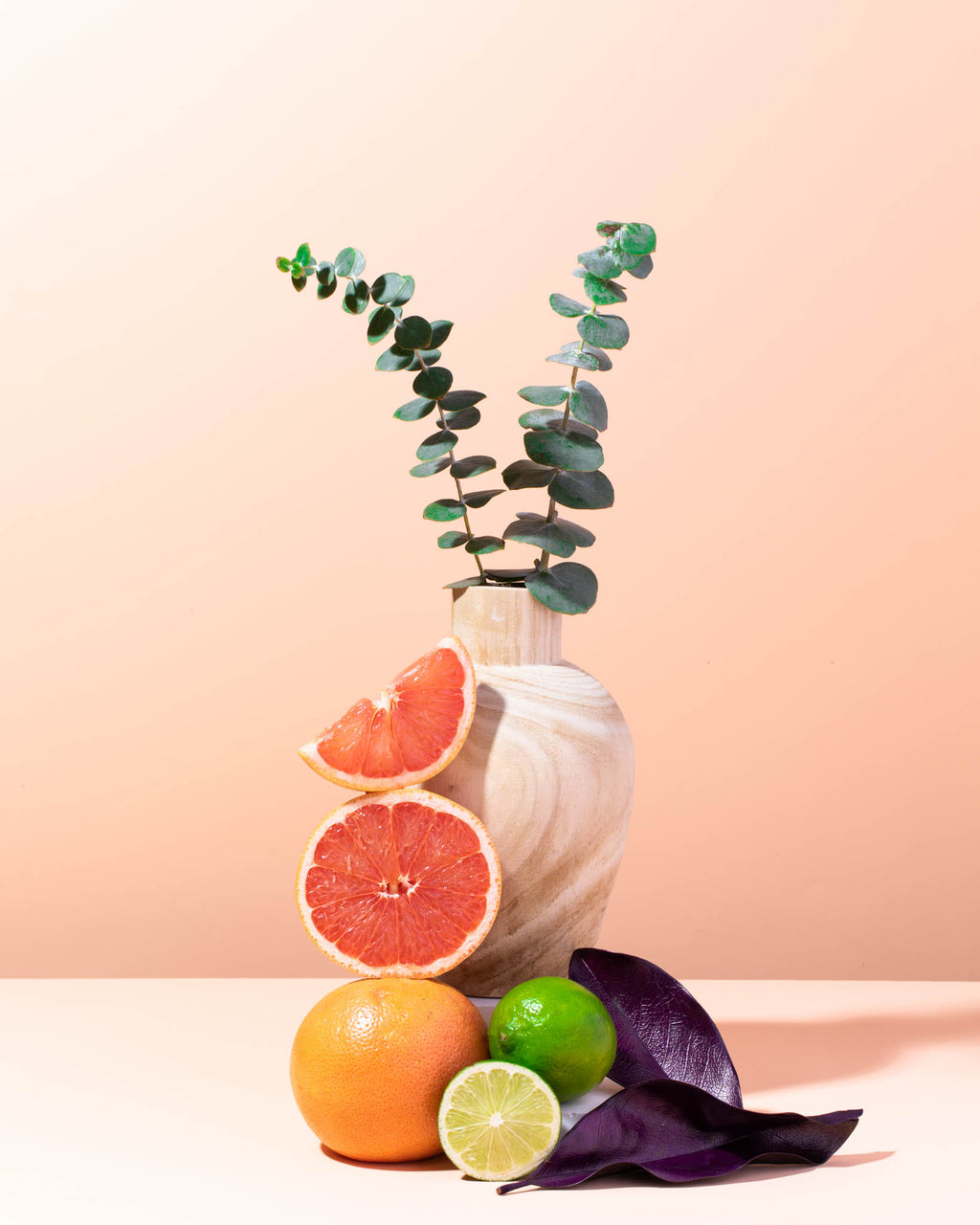In this meticulously staged, vertically rectangular photograph, vibrant fruit and foliage are artfully arranged against a soft pink backdrop under artificial lighting. Anchoring the composition is a white vase containing two sprigs of upright eucalyptus. To the right of the vase, a striking fruit tower begins with a full orange at the base, topped sequentially by a half and then a quarter pink grapefruit slice. Adjacent to this stack is a whole lime with a cut lime wedge positioned in front of it. Adding a splash of contrast, two dark purple leaves lay beside the lime. The scene is set on a surface that transitions to a lighter pink, casting a clear shadow from the vase. This captivating assembly, devoid of text, emanates a sophisticated yet playful vibe, showcasing a harmonious blend of greens, pinks, oranges, purples, and beige tones.